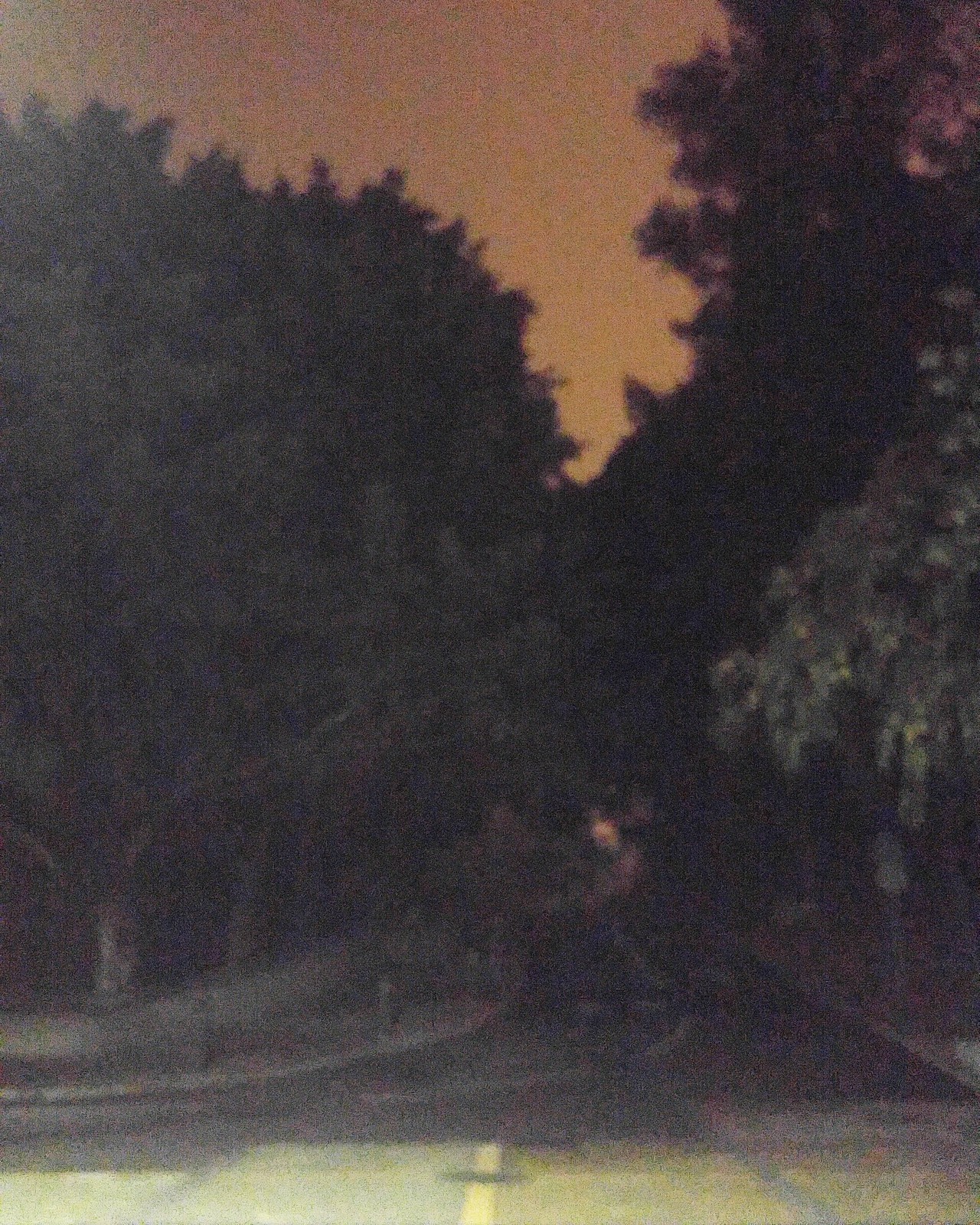This nighttime photograph captures a surreal scene where an orange-hued sky serves as a dramatic backdrop. The image, though slightly out of focus, reveals a winding road bordered by a concrete wall. Street poles punctuate the roadside, and the foreground features what appears to be a crosswalk, delineated by faint, stripe-like patterns. The silhouettes of approximately ten trees are discernible, adding a touch of eerie beauty to the frame as they stand against the glowing sky.